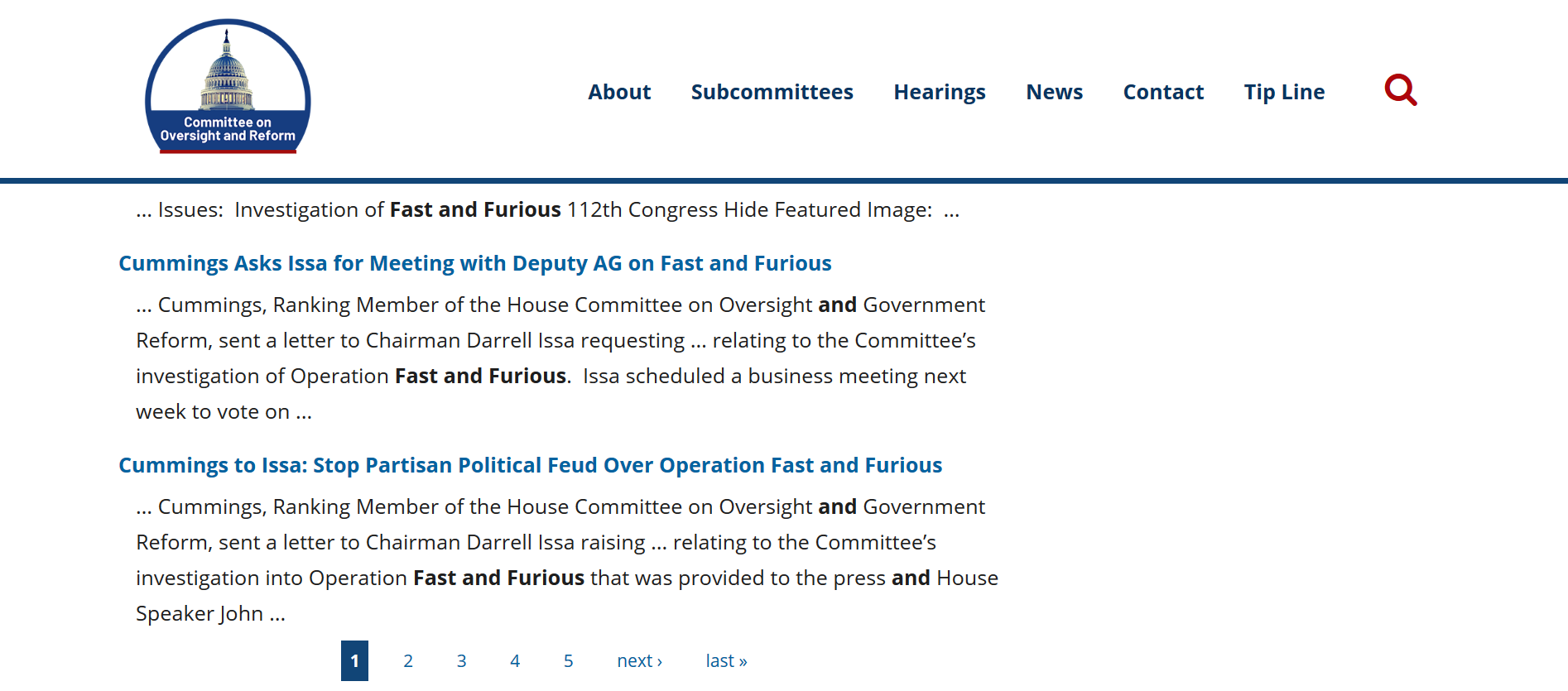This is a detailed screenshot of the website for the Committee on Oversight and Reform. The layout includes a white background in the top-left corner showcasing a logo featuring a photograph of the Capitol building's dome encased in a blue snow globe outline. Beneath the logo, a dark blue band displays the text "Committee on Oversight and Reform" in white. 

A thin dark gray line runs below this band. To the right, separated by some negative space, are navigation links in black text labeled "About," "Subcommittees," "Hearings," "News," "Contact," and "Tip line." Adjacent to these links, a dark red magnifying glass icon signifies the search function.

Below the main header, a medium-width dark blue line stretches across the entire page width. The body of the page begins with a line of black text that reads, "Issues: Investigation of Fast and Furious 112th Congress. Hide Featured Image:" 

Following this, in blue text, it states, "Cummings asks ISSA for a meeting with Deputy AG on Fast and Furious." 

Next is a black text paragraph summarizing the news: "Cummings, Ranking Member of the House Committee on Oversight and Government Reform, sent a letter to Chairman Darrell ISSA requesting... Relating to the Committee's Investigation of Operation Fast and Furious, ISSA scheduled a business meeting next week to vote on..." This is followed by another line of unspecified blue text.